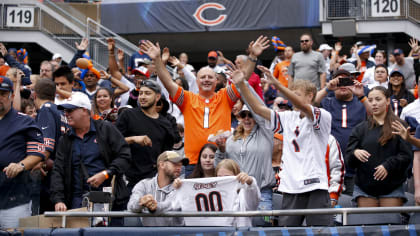The image depicts a vibrant scene of spectators at a sporting event, likely a Cubs game, suggested by the vibrant orange "C" emblem with a white outline on a blue background. Central to the photograph is an older bald man wearing a fluorescent orange shirt with a white line down the center, standing with arms lifted high and a broad smile directed at the camera. Surrounding him is a diverse crowd of excited fans, both men and women, also raising their hands in enthusiasm. Notably, a woman among them is prominently holding up a white jersey marked with the number 00. The scene is framed by the stadium sections numbered 119 on the left and 120 on the right, firmly anchoring the image in the energetic atmosphere of a live sports event.